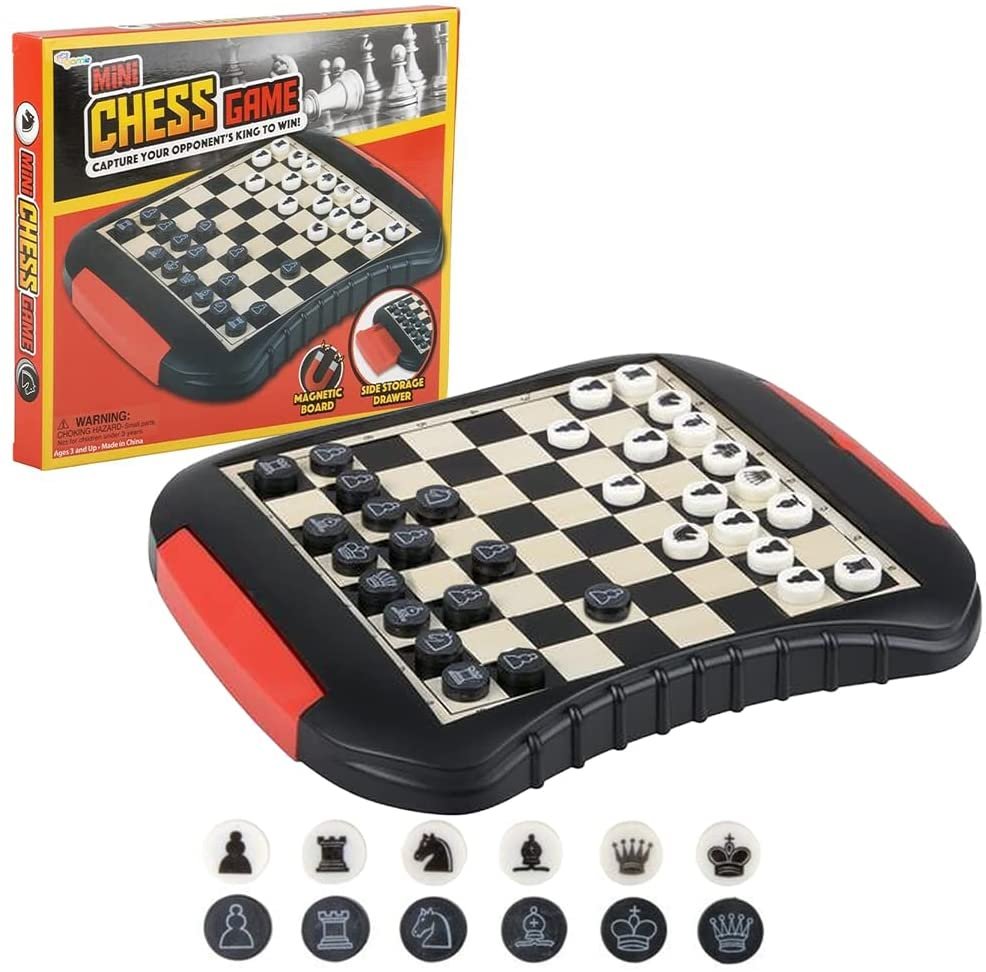The image showcases a Mini Chess Game set against a white background. Dominating the top left is a rectangular game box, predominantly red with yellow highlighting around its edges. The box features the tagline "Mini Chess Game - Capture Your Opponent's King to Win," and prominently displays a black plastic chess board with a checkerboard pattern. This board is flanked by red storage shelves for the pieces. Unique to this set, the chess pieces are circular discs, with black pieces bearing white-outlined symbols and white pieces sporting solid black icons representing traditional chess figures such as kings, queens, knights, and rooks. The game is described as magnetic for convenience.